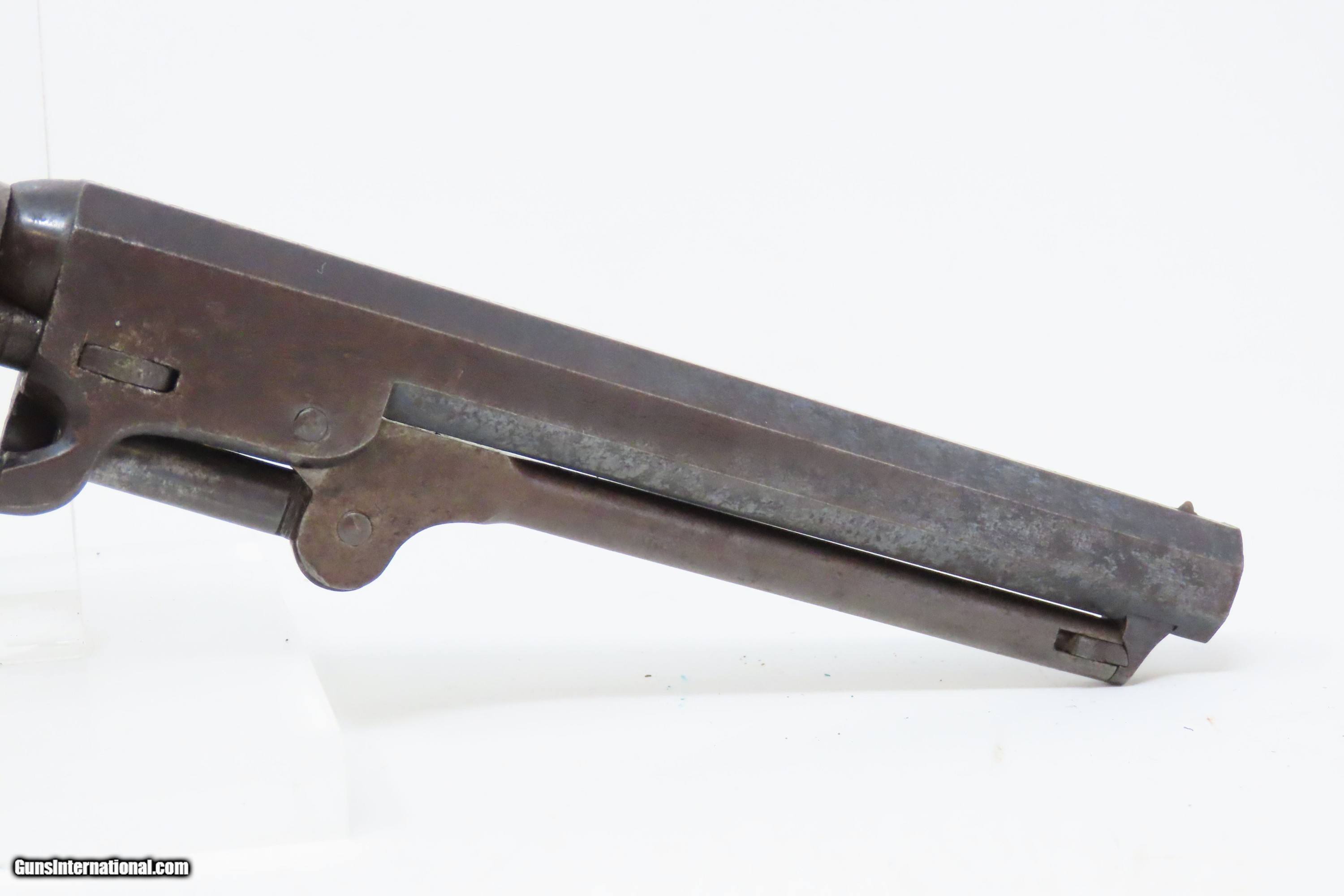This image depicts a side view of the barrel of an antique or vintage gun resting on a white background. The metallic surface of the barrel shows significant signs of erosion and rust, giving it a distinctive brownish-red hue in some areas, while other parts reveal the bare gray metal. The front portion of the gun is placed on a white surface, with the back end slightly elevated. The barrel itself appears to be around a foot long, suggesting it might belong to a sawed-off shotgun or a similar firearm. In the bottom left corner of the image, there is text that reads "gunsinternational.com," outlined in black. 

By incorporating details from each caption, the description emphasizes the gun's old and rusty appearance, the visible segment of the barrel, and specific elements such as the background and the text included in the image.